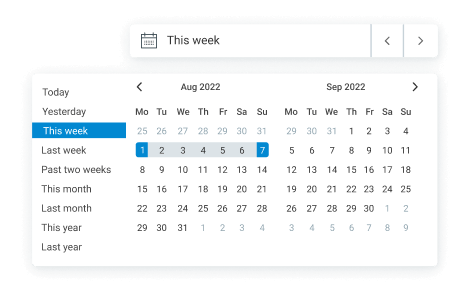In the image, a detailed vector graphic of a calendar interface is presented. At the top left, there's an icon resembling a hanging calendar. To its right, the term "This Week" is prominently displayed. Adjacent to this text are two navigation arrows: one pointing left and the other pointing right.

Directly below, the left-hand column lists various time periods such as "Today," "Yesterday," "This Week," "Last Week," "Past Two Weeks," "This Month," "Last Month," and "Last Year." Highlighted in this column is "This Week."

To the right of this column, two more columns feature individual calendars. Above the first calendar, the text "August 2022" is displayed with a left-pointing arrow beside it. In the adjacent column, the second calendar is titled "September 2022" with a right-pointing arrow.

Both calendars display the dates from the 1st to the 7th of their respective months. In the left calendar, highlighting marks the dates from Monday, the 1st to Sunday, the 7th, using a distinctive blue background. The numbers within these dates are black, and the background for the remaining dates is a light gray.